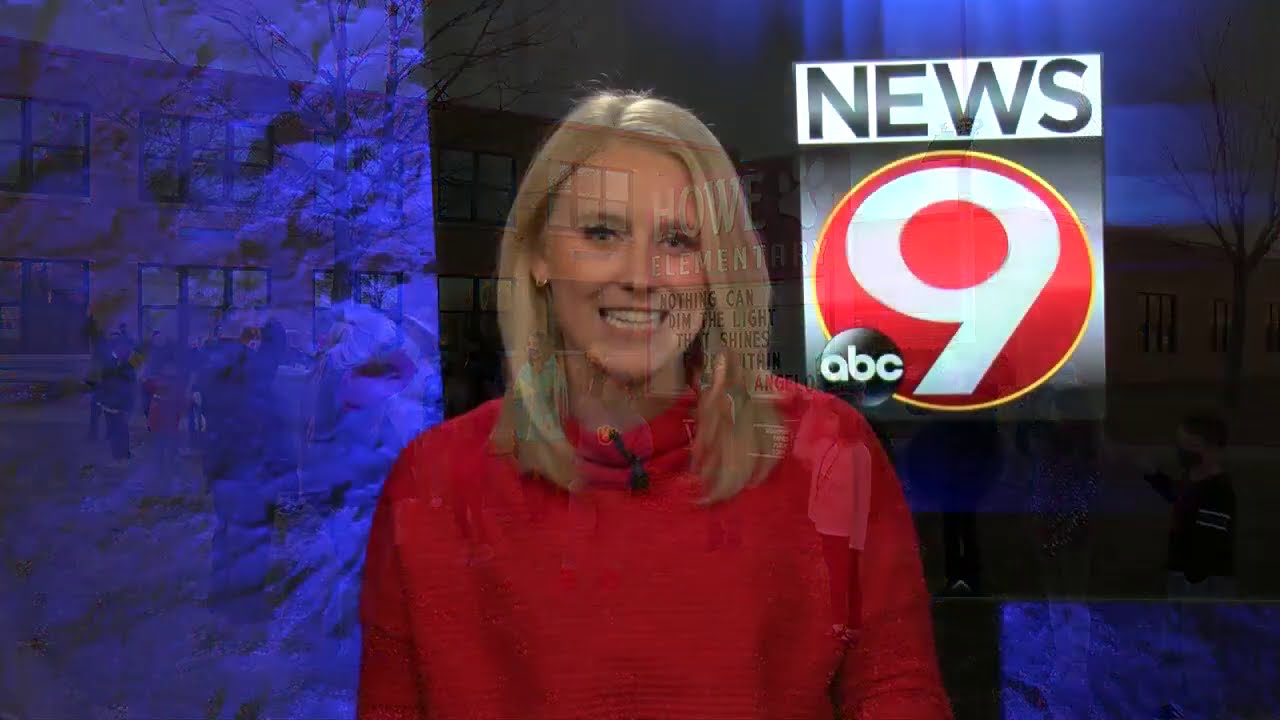This image is a screen capture from a News 9 ABC broadcast, featuring a blonde-haired, white female news anchor with dark eyes at its center. She is smiling and talking, revealing her teeth, while wearing a red turtleneck blouse with a microphone clipped to the front. The background is layered and visually intriguing, combining a blurred, purple-blue backdrop with a superimposed image of Howe Elementary School. This superimposed image shows a building with people, possibly students, standing in the parking lot in front of it. To the news anchor’s right, positioned just above her shoulder, is the News 9 ABC logo, which features the word "News" in black letters on a white background, with a red circle enclosing the number "9" below it, and the letters "ABC" positioned at the bottom. Additionally, text on the left of the background reads “Howe Elementary,” followed by a partially visible slogan: "Nothing can dim the light that shines..." The vivid detail of the scene effectively combines the professional demeanor of the news anchor with the subtle hints of the informative story being covered.